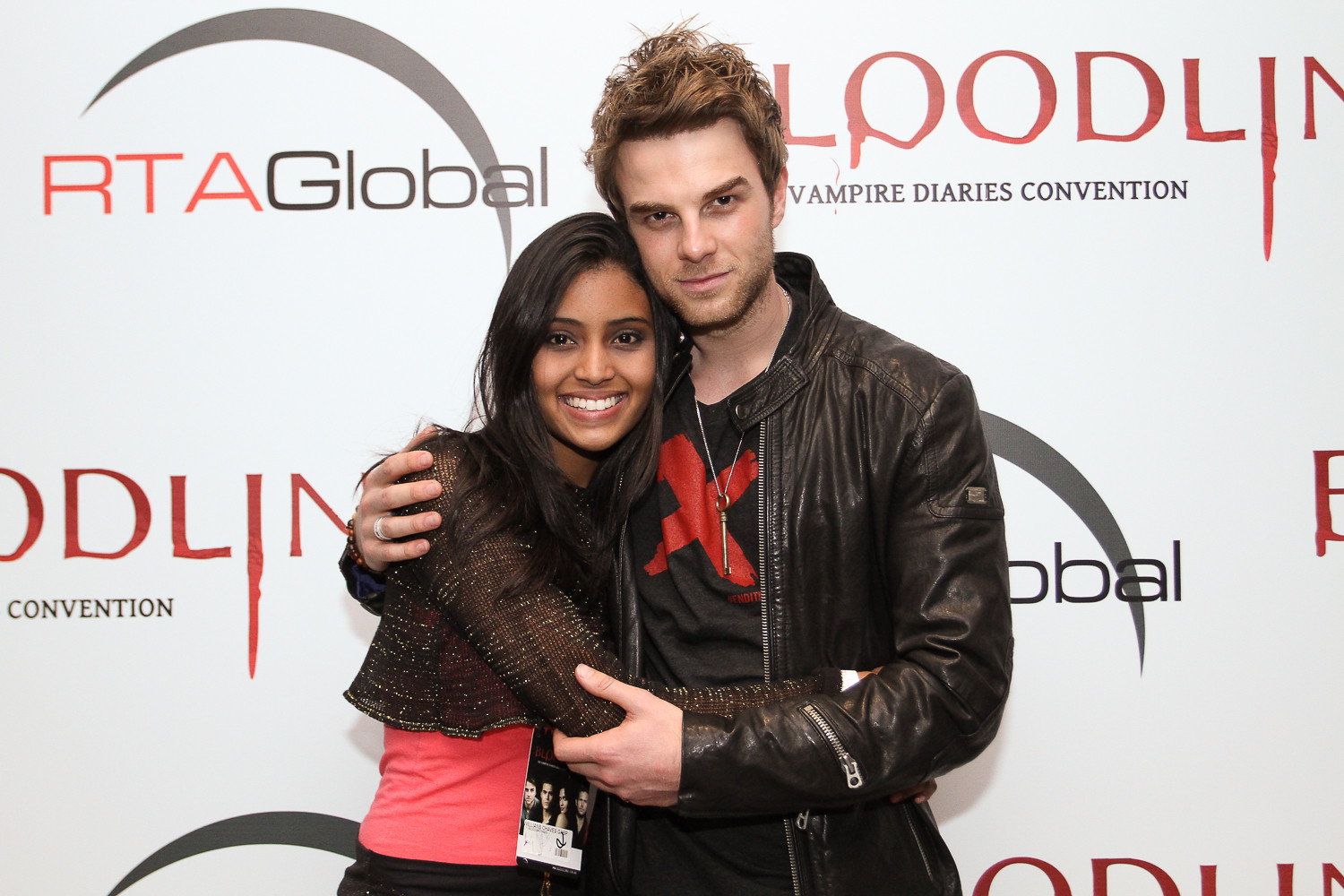In this image, a young white male, approximately 18 to 22 years old, and an African-American light-skinned female are posed in front of a white banner. The woman wears a cropped, brown spotty top and black pants, while the man sports a leather jacket with a distinctive red X and scraggly hair, giving him a somewhat menacing look. His right arm is draped around the woman's shoulder, suggesting a warm embrace, while she smiles brightly at the camera. A press pass hangs around her neck. The banner behind them prominently features the text "Bloodline Vampire Diaries Convention" in red and black, as well as "RTA Global" in orange and black, against a backdrop with a half-moon symbol. The couple appears to be attending this convention, and they are centered in the image, clearly the focus without any other visible objects or readable text around them. The overall setting suggests an indoor event, likely a fan convention.